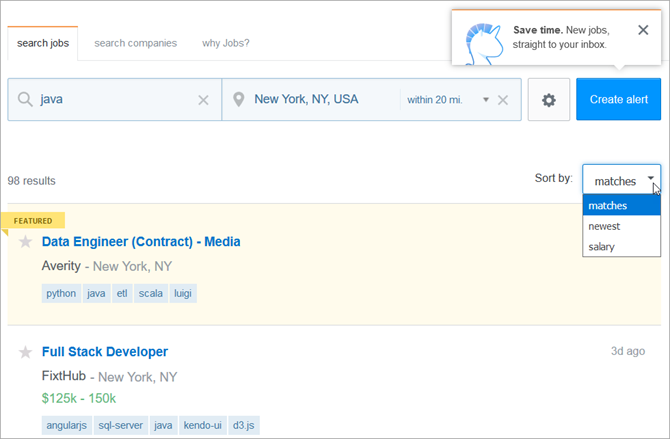This image depicts a computer screen displaying a job search webpage. At the top of the page, there's a tab labeled "Search Jobs." In the search bar, the user has typed "Java," and a pinned location note indicates "New York, NY, USA" with a search radius of "within 20 miles." Below this, one job listing stands out with a banner titled "Featured," indicating a position for a "Data Engineer - Contract - Media."

Scrolling down, another job listing appears for a "Full Stack Developer" at a company called "Fix Hub," offering a salary range of $125,000 to $150,000. Additionally, a cartoon drawing of a unicorn (lacking visible eyes but featuring a horn) is prominent at the top, accompanied by text that reads, "Save time, new jobs straight to your inbox." Next to this graphic is a blue clickable button labeled "Create Alert."

Towards the top-right corner, there's a dropdown menu offering sorting options: "Matches," "Newest," and "Salary," with "Matches" currently selected.